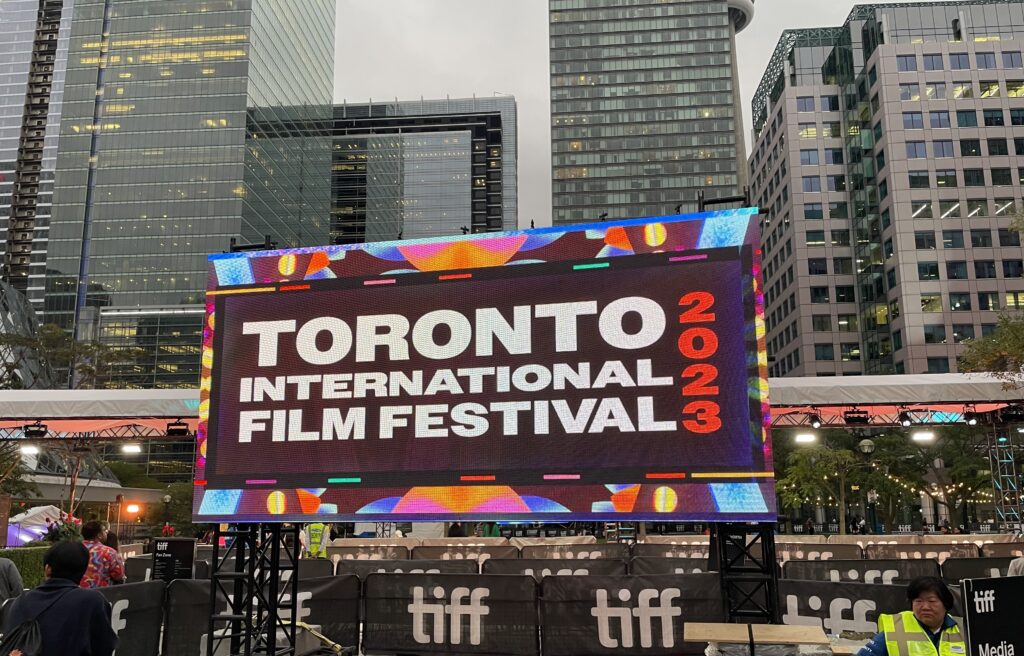In this vibrant photograph taken at the Toronto International Film Festival of 2023, the scene is dominated by a large, colorful banner that prominently displays "Toronto International Film Festival" in white lettering, accompanied by "2023" in bold red text running vertically. The sign itself is surrounded by a brightly lit billboard, enhancing the celebratory atmosphere with hues of blue, yellow, pink, and orange. The backdrop reveals a cityscape punctuated by tall, mostly glass buildings, aglow with lights, suggesting the photo was captured around dusk. A queue area is visible in the foreground, though currently empty of people, and positioned at the bottom right is a security guard in a neon yellow vest, ensuring the area remains secure as preparations for the festival continue. The overall scene exudes anticipation and readiness for the grand event to commence.